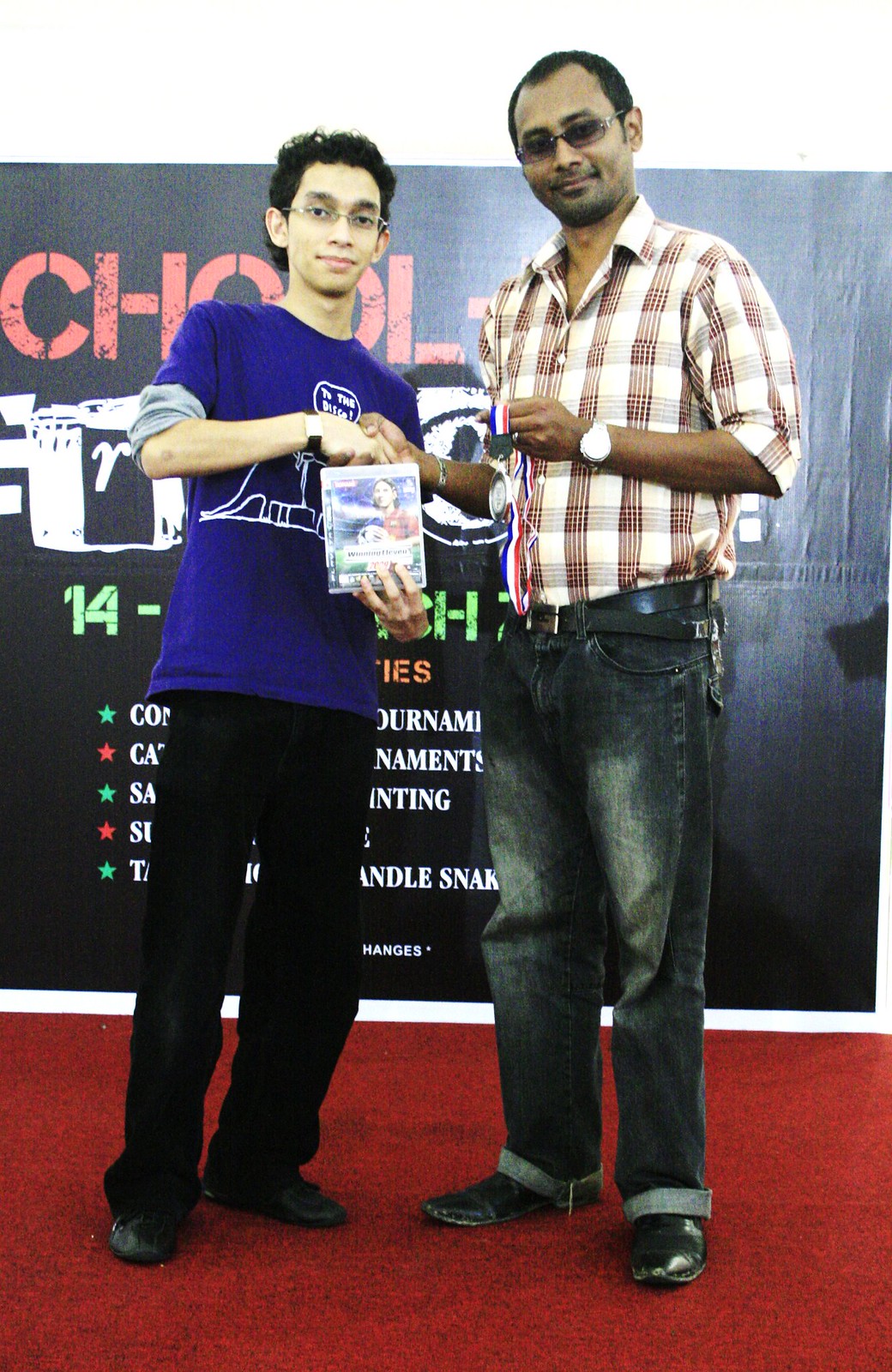In the image, a pre-teen boy with curly hair, glasses, and a watch on his wrist is shaking hands with an older man. The young boy, standing on the left, wears a blue short-sleeve t-shirt featuring a cartoon dinosaur design, black pants, and black shoes. He's holding what appears to be a video game case in his left hand. Opposite him, the older man on the right, also wearing glasses and a watch, is dressed in a plaid red and white short-sleeve button-down shirt and blue jeans with a belt. He is handing the boy a red, white, and blue ribbon with a medallion attached. Both are standing on a red carpet in front of a dark wall with unreadable text.